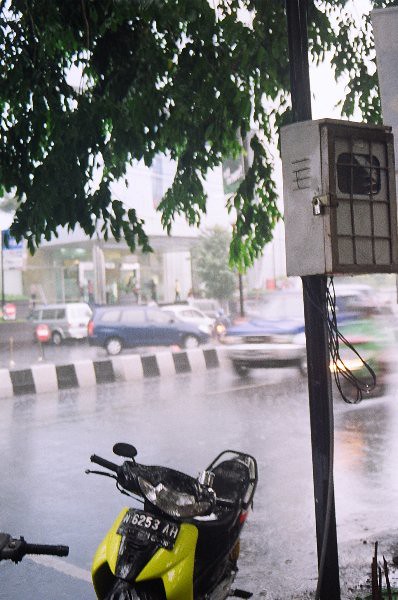In this detailed photograph taken outdoors during a heavy downpour, the scene captures a sopping wet pavement indicative of the rainy day's intensity. Centered in the foreground is a primarily green motorbike with a black frame, bearing a license plate reading N62538H. To the right of the motorbike, a tall black pole stands, equipped with a rectangular metal box attached to it, possibly a secured lockbox. Just beside it, the handle of another scooter, yellow in color, slightly peeks into view from the lower left corner of the image. Overarching branches and leaves, suggesting that the photo was taken from under a tree, frame the top part of the composition. In the background, cars can be seen both parked and in motion on the road, with a blurred blue car moving diagonally towards the photographer. Beyond the street, a white and black barrier separates the road from a business center and additional parked vehicles, with a building and a few pedestrians seeking cover visible in the distance. The overall gray ambiance of the day, coupled with the blurred movement of the traffic, emphasizes the heavy rain and the bustling yet soaked urban environment.